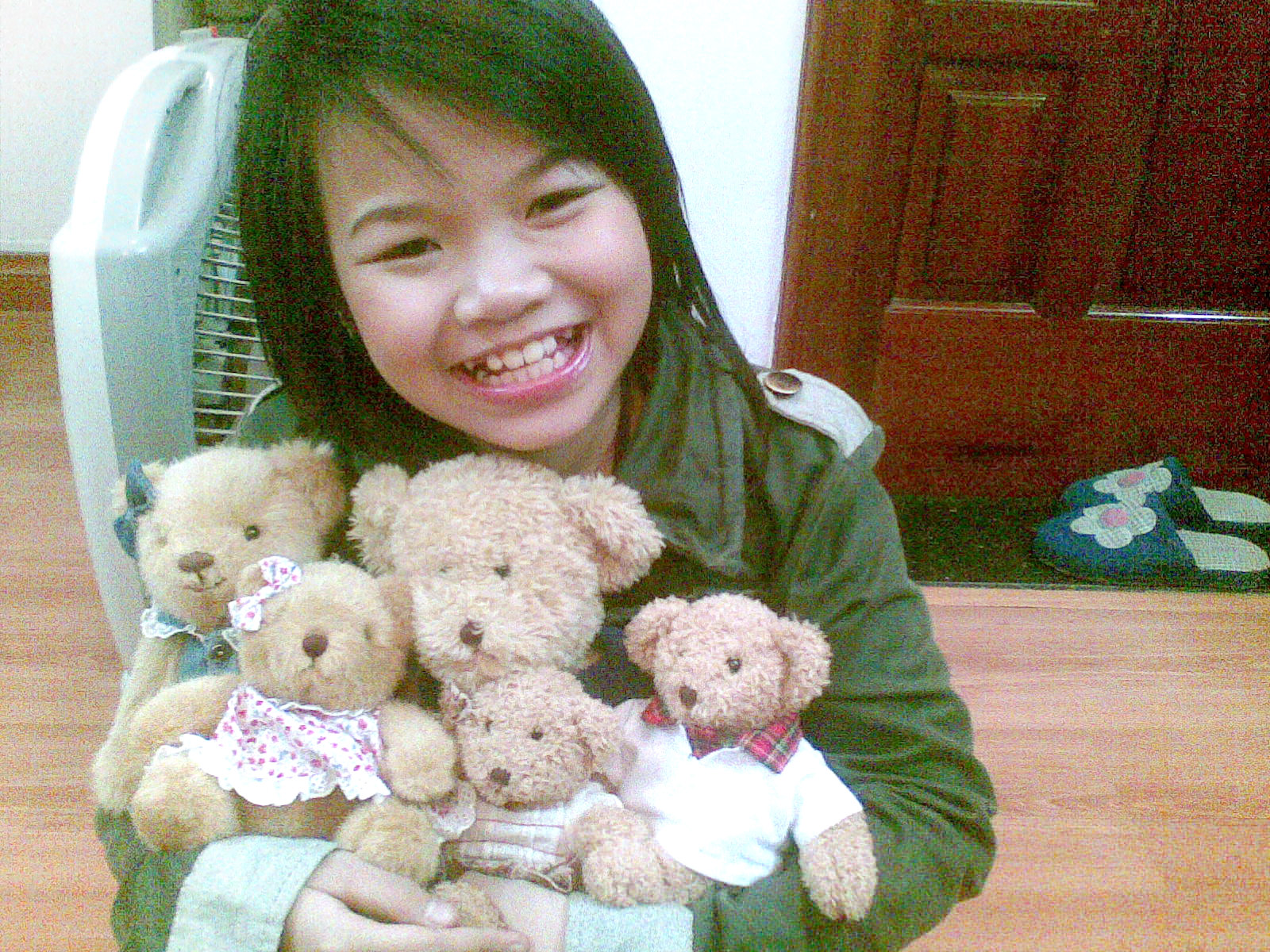In the photograph, we see a young Asian girl, likely around seven or eight years old, radiating joy with a large smile on her face. She has dark hair that cascades to her shoulders and delicately arched eyebrows. Dressed in a forest green coat with white lapels and gold buttons, she stands confidently, holding a close-knit family of five teddy bears. Each bear, varying in size, is dressed distinctively—one bear sports a white bow with pink flowers and a matching dress, another has a white shirt with a red plaid collar, while others wear green bows and dresses.

The background features a dark brown wooden door with a pair of teal slippers adorned with white petals and pink centers resting on a dark green throw rug. The light wooden floor adds warmth to the setting, complementing the scene. To the left of the girl, a silver or gray fan sits on the floor, hinting at the family's attention to comfort.

The photograph captures a beautifully nuanced moment of innocence and happiness, framed by the inviting ambiance of a homely, well-kept interior.